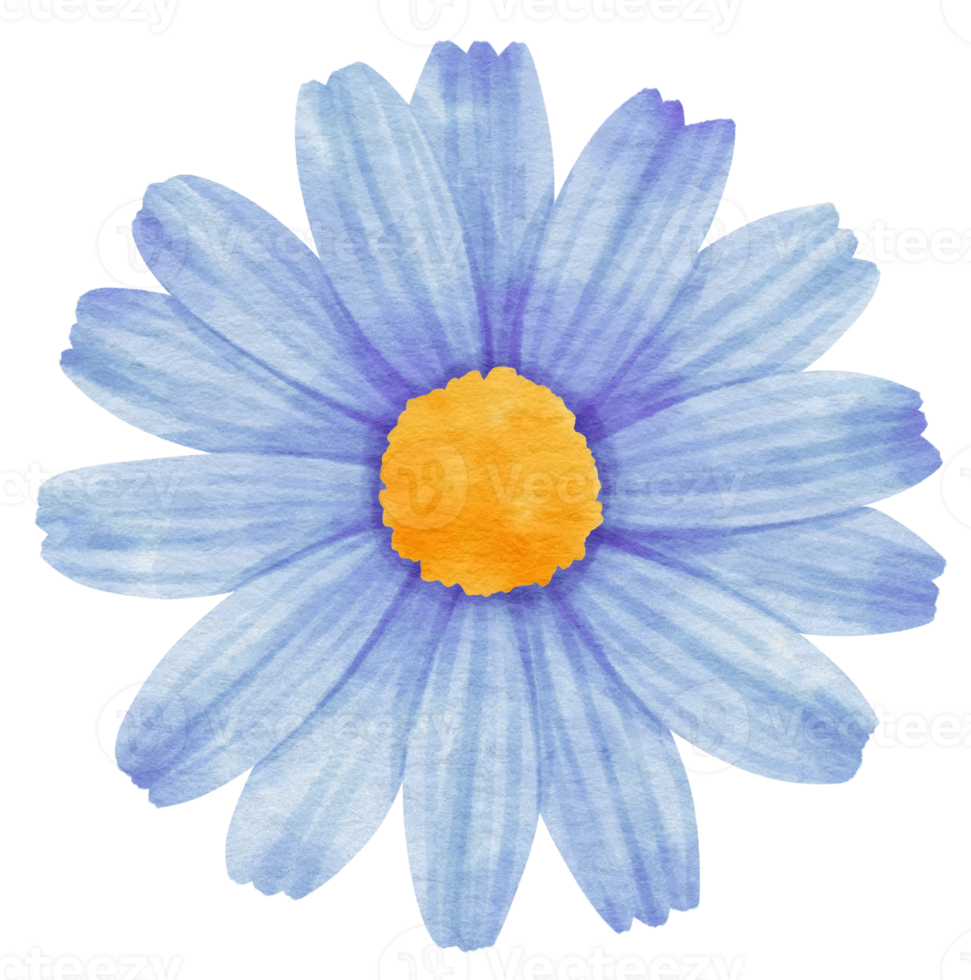This artist's rendering features a detailed watercolor portrayal of a blue daisy prominently centered against a white background. The daisy exhibits elongated, oval-shaped petals that transition from a violet-blue near the base to a lighter bluish hue towards the tips, with a resurgence of deeper color at the ends, which are uniquely jagged. A vibrant, gradient yellow-to-orange center sits at the heart of the flower, enhancing its captivating aesthetic. The image carries a faint watermark reading "Vecteezy," repeated in low opacity across the painting. With no artist signature or extraneous elements, the focus remains solely on the striking, multifaceted petals and the strong, warm-toned core of the flower.